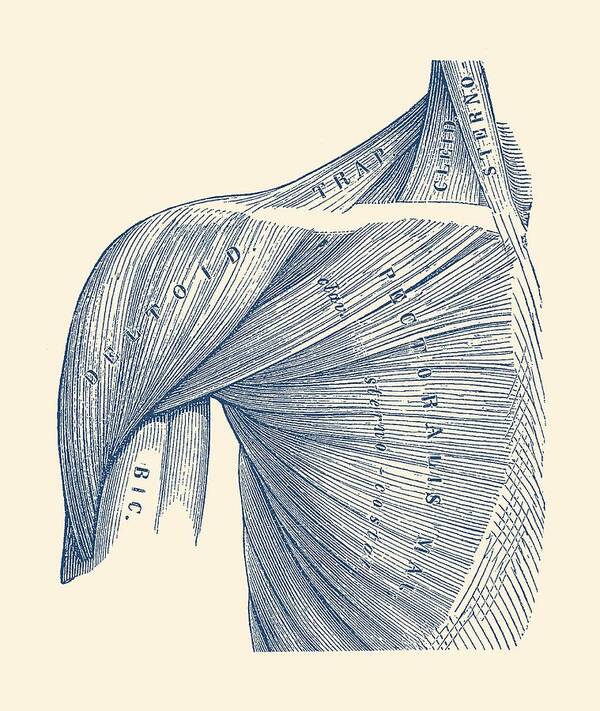This detailed illustration resembles a meticulous pencil sketch one might encounter in a biology textbook, portraying the right shoulder and upper torso muscles. The background features a soft, off-yellow hue, enhancing the clarity of the black and white pencil details. Prominent muscle groups such as the deltoid, labeled in light blue text, the trapezoid, marked as "TRAP," and various other muscles, are vividly depicted with intricate lines indicating the direction of the muscle fibers. The labels, rendered in similar blue text, add a layer of educational value to the illustration, guiding the viewer's understanding of the anatomical features. The meticulous rendering focuses primarily on the deltoid, trapezoid, and pectorals, excluding the arm muscles and anything below the pectorals, providing a concentrated study of this section of human anatomy.